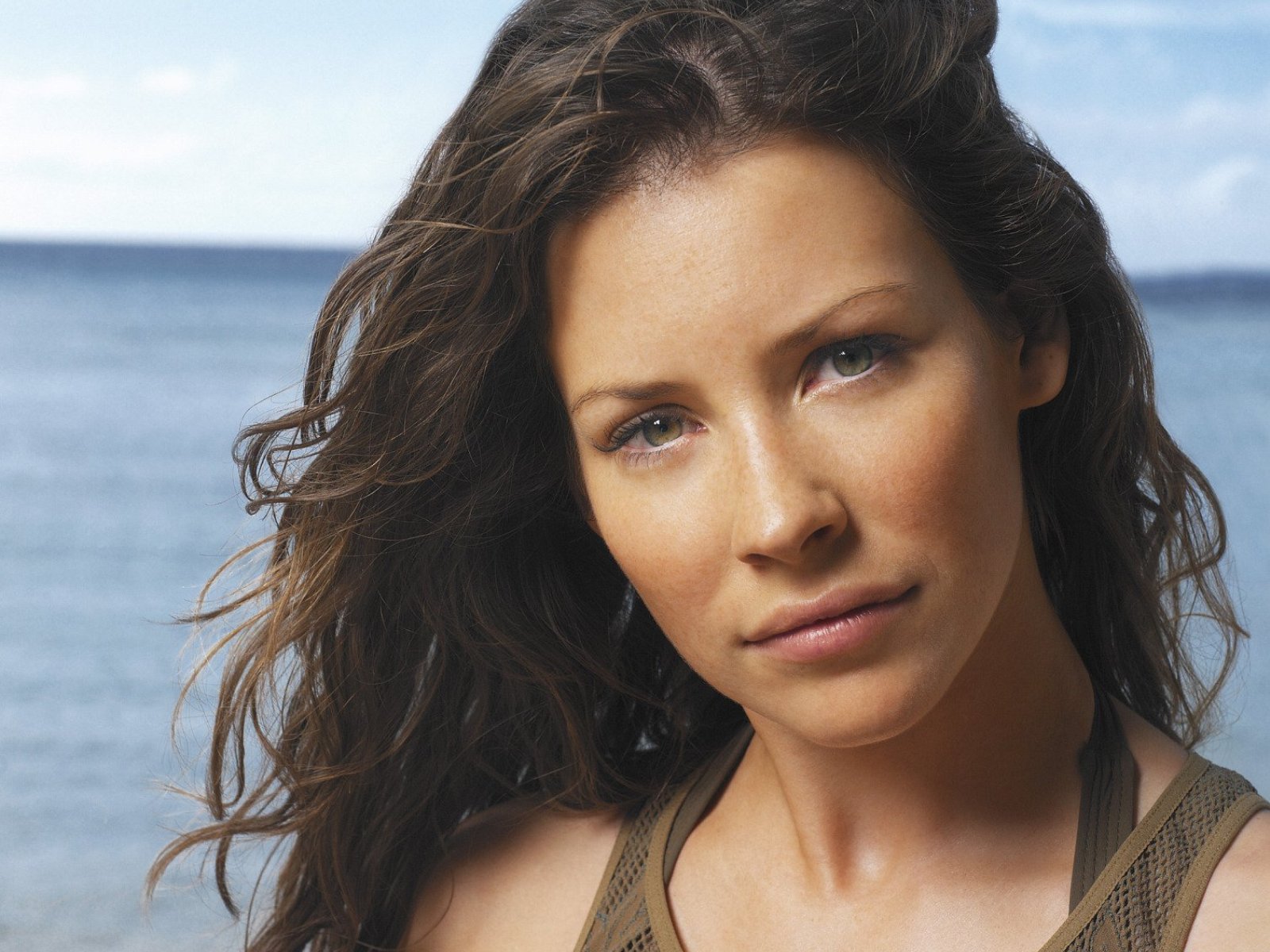In this image, we see a detailed outdoor scene set on a beach during the day. At the center of the composition is actress Evangeline Lilly, famously known for her role in the show "Lost." The photograph appears to be a promotional shot from the series. Lilly is captured from the shoulders up, her gaze directed at the camera. She has slightly frizzy, dark hair with lighter tips, styled with a light curl that sweeps over to one side. She is wearing a brown mesh tank top layered over a brown bra, with no visible text in the image. The background features a large body of water that appears lighter near the foreground and darker toward the horizon. Above, a hazy blue sky with a few scattered clouds adds a subtle contrast. The color palette includes light blue, white, gray, black, tan, brown, pink, and olive, evoking a serene, natural ambiance often associated with beach settings.